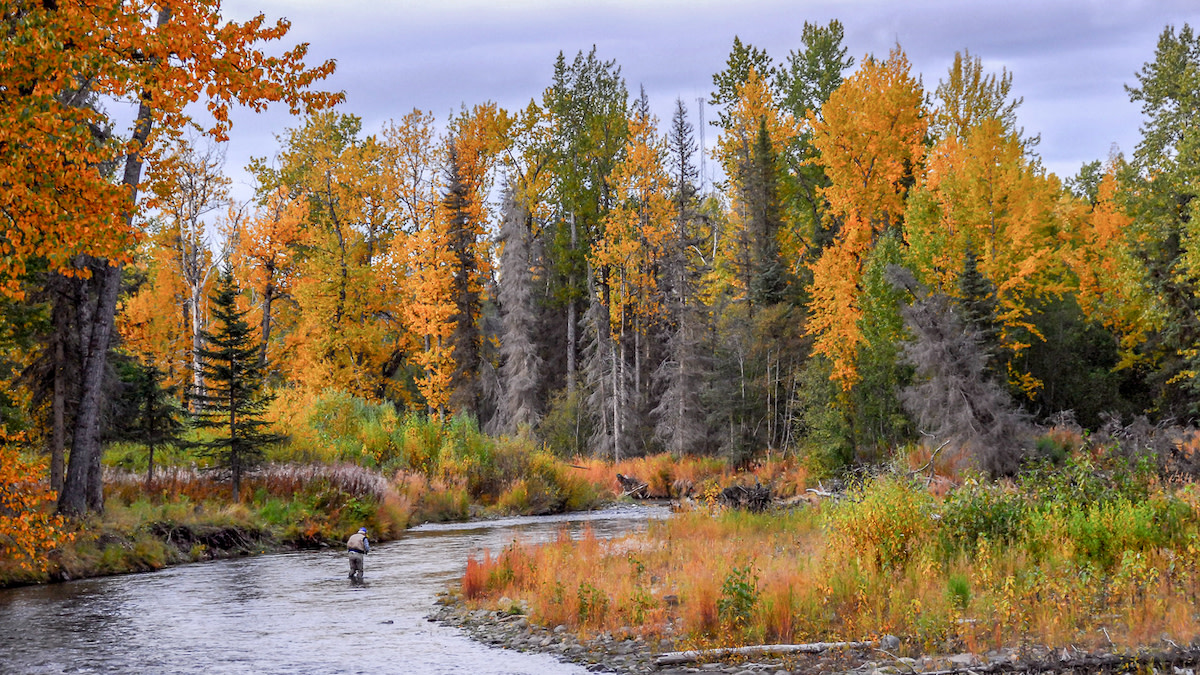This vivid color photograph captures a picturesque outdoor scene in the fall. Dominating the image is a winding, calm river stretching from the left to the right side of the frame. Central to the river is a figure of a person, clad in dark waders, a khaki vest over a blue long-sleeve shirt, gray pants, and a blue cap, with a hint of gray hair visible. The person appears to be fishing, although the fishing rod is faint and hard to discern. The riverbank on both sides features a lush display of fall foliage, with grasses and bushes gleaming in vibrant hues of orange, red, yellow, and lingering greens. On the right riverbank, a smattering of small rocks and pebbles leads to a beautiful blend of multicolored grasses. The left riverbank boasts a striking tree with orange leaves standing tall beside a small pine tree. The background is framed by a diverse tree line, some trees bare or grayish, others adorned in their seasonal reds, oranges, and greens. The serene sky above completes this tranquil autumnal landscape, evoking a sense of peaceful solitude amidst nature's seasonal splendor.